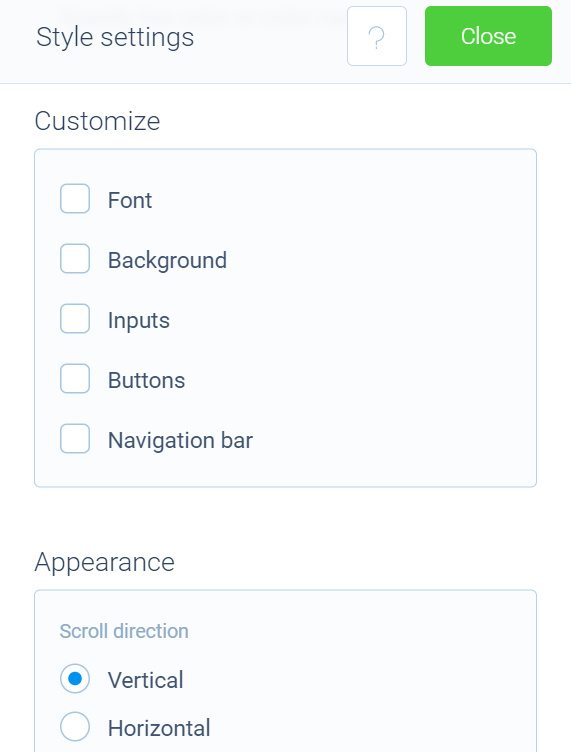The image displays the settings interface of a mobile application, shown in portrait orientation without distinct borders. At the top, a prominent horizontal rectangle serves as a header. On the left side of this header, there's the label "Style Settings," accompanied by a white square with a blue outline and a blue question mark inside. Adjacent to this, a long, green, rounded rectangular button with white text reads "Close."

Below this header lies a section of white space followed by a black "Customize" header. Beneath this header, nestled in a grey rectangle with a blue border, are five customizable options: Font, Background, Inputs, Buttons, and Navigation Bars. Each option is paired with a square checkbox featuring rounded edges, white interiors, and blue borders, although none are checked.

Further down, there's additional white space and a title labeled "Appearance." This is followed by another gray rectangle with a blue border containing a subheader in gray text that says "Scroll Direction." Within this section, there are two options: Vertical and Horizontal, each with a corresponding radio button. The radio button next to Vertical is selected, indicated by a filled blue circle.